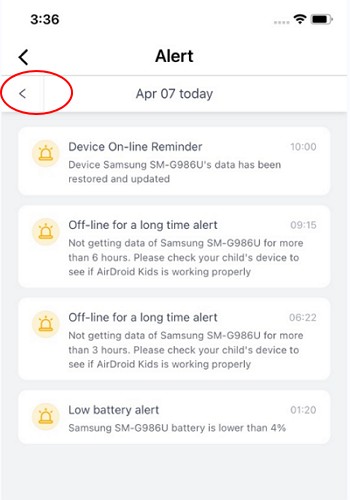The image showcases a smartphone screen displaying an alert notification at precisely 3:36 PM, with the battery level indicating approximately 90% charge. At the top of the screen, the date is marked as April 7th (APR07), labeled as "Today." A manually drawn red circle highlights the back button, suggesting the user can navigate to a different date.

The primary alert heading, "Device Online Reminder," is prominently displayed in a dark color, with an accompanying arrow pointing to the left. Below this heading, the notification details a specific device, a Samsung model, whose data has been restored and updated at 10:00 AM.

Following this, in a white rectangle, there's another alert titled "Offline for a long time alert." It indicates that the Samsung device has not been sending data for more than six hours. The message urges the user to check if the AirDroid Kids application on their child's device is functioning correctly.

Additionally, the screen features two more alert messages, each accompanied by a small, yellow alert bell icon on the left side.